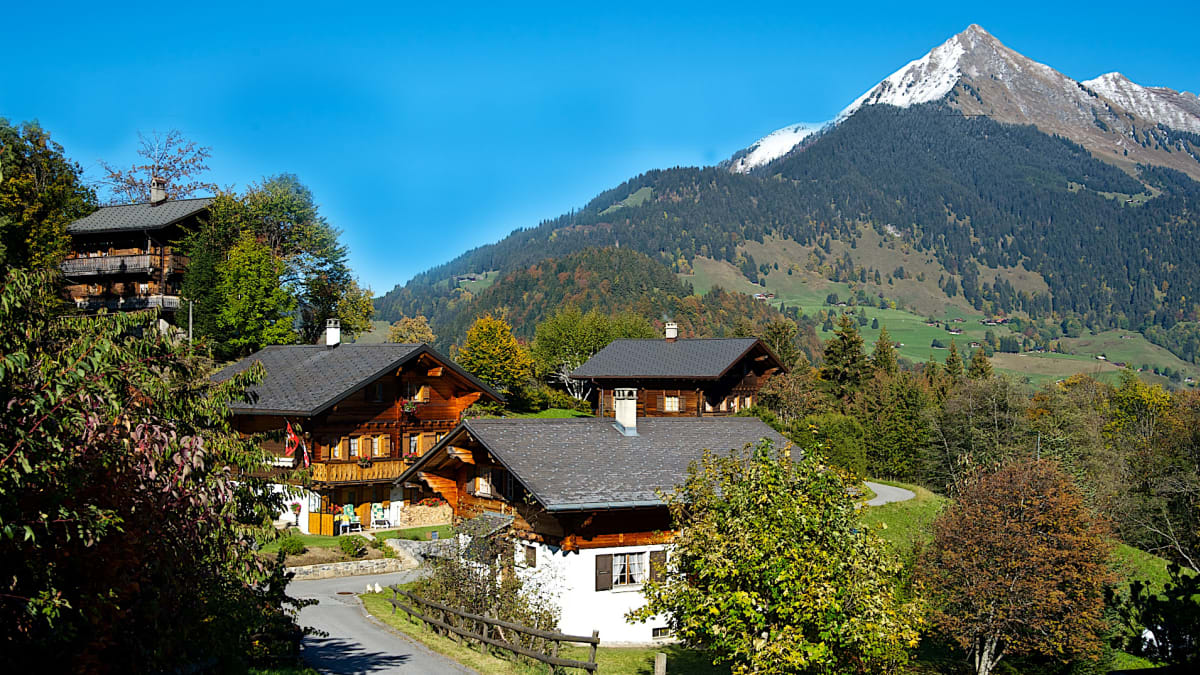The image captures a picturesque village nestled high in the mountains, reminiscent of a serene getaway in the Swiss Alps. The background features a towering, majestic mountain with snow-capped gray peaks and lush trees cascading down its slopes. Under a bright blue, cloudless sky, the sun illuminates the verdant green fields and rolling hills that frame the scene. 

At the village's base, four distinct, cabin-like houses sit along a road. To the left is a two-story house perched higher than the others, featuring a gray roof, white chimney, and a balcony encircling the top story. Its immediate neighbor also has two stories, a similar balcony, and a red flag hanging from it. Further right stands a smaller white house with an awning over one window and a brown fence running parallel to the road. The final house in the row is made of brown wood with a gray roof, completing the quartet with a backdrop of stately trees and inviting green yards.

The village exudes a peaceful, welcoming atmosphere, with its earth-toned houses, expansive green spaces, and mountain vistas offering a picturesque retreat from the hustle and bustle of city life.